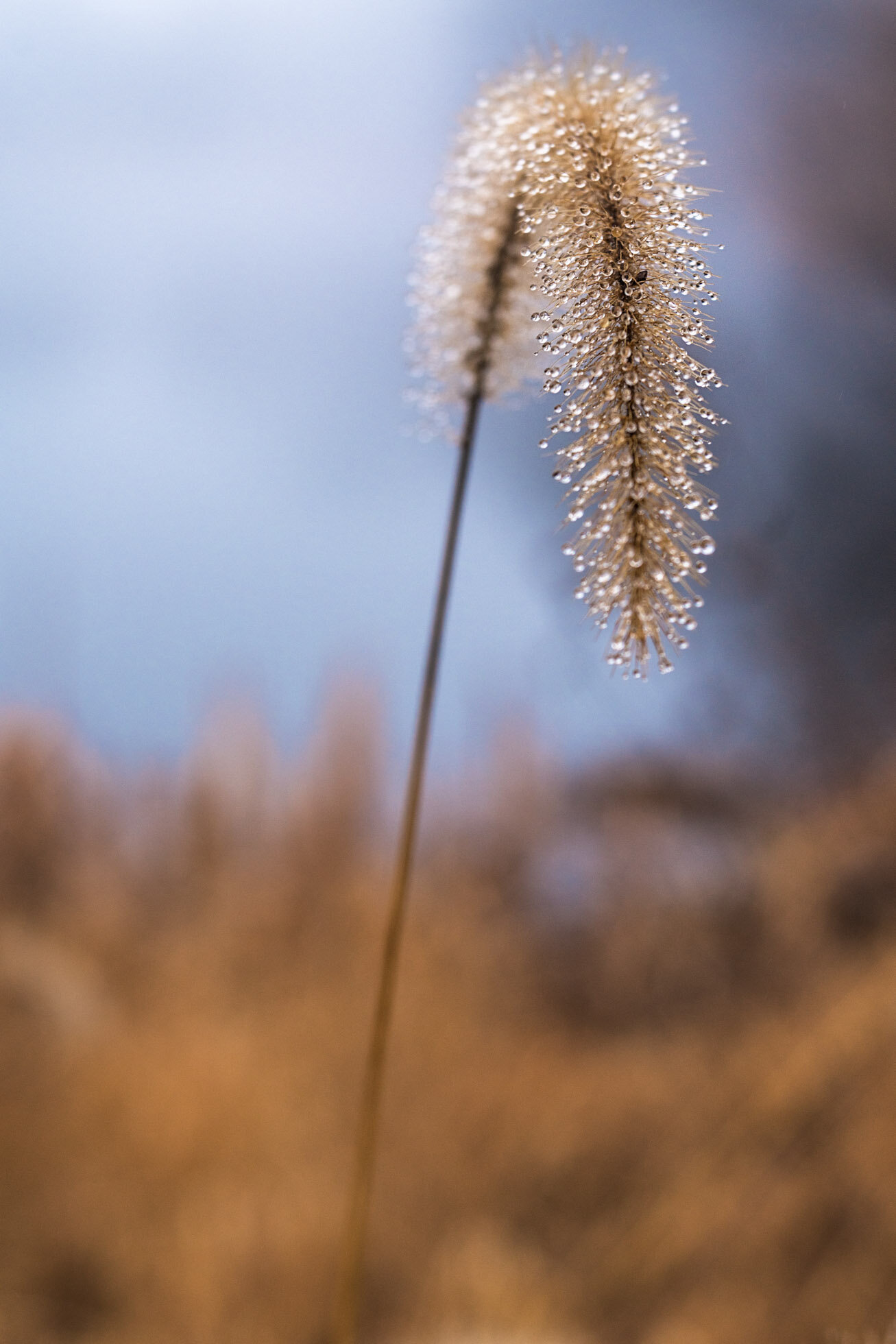This image captures a close-up of a solitary cattail plant, prominently bent into an arch or U-shape due to the weight of numerous water droplets on its fuzzy, light silver fluff. With a thin, long, brown stem, this cattail shows the signs of being at the end of its season, indicated by its beige and somewhat weathered appearance. The background is entirely out of focus, offering a mix of blurred ground that is brown and what hints at a field of similar plants under a softly blurred blue sky. The absence of people, animals, or insects directs all attention to the solitary, dew-laden cattail, evocatively reminiscent of childhood memories of outdoor play.